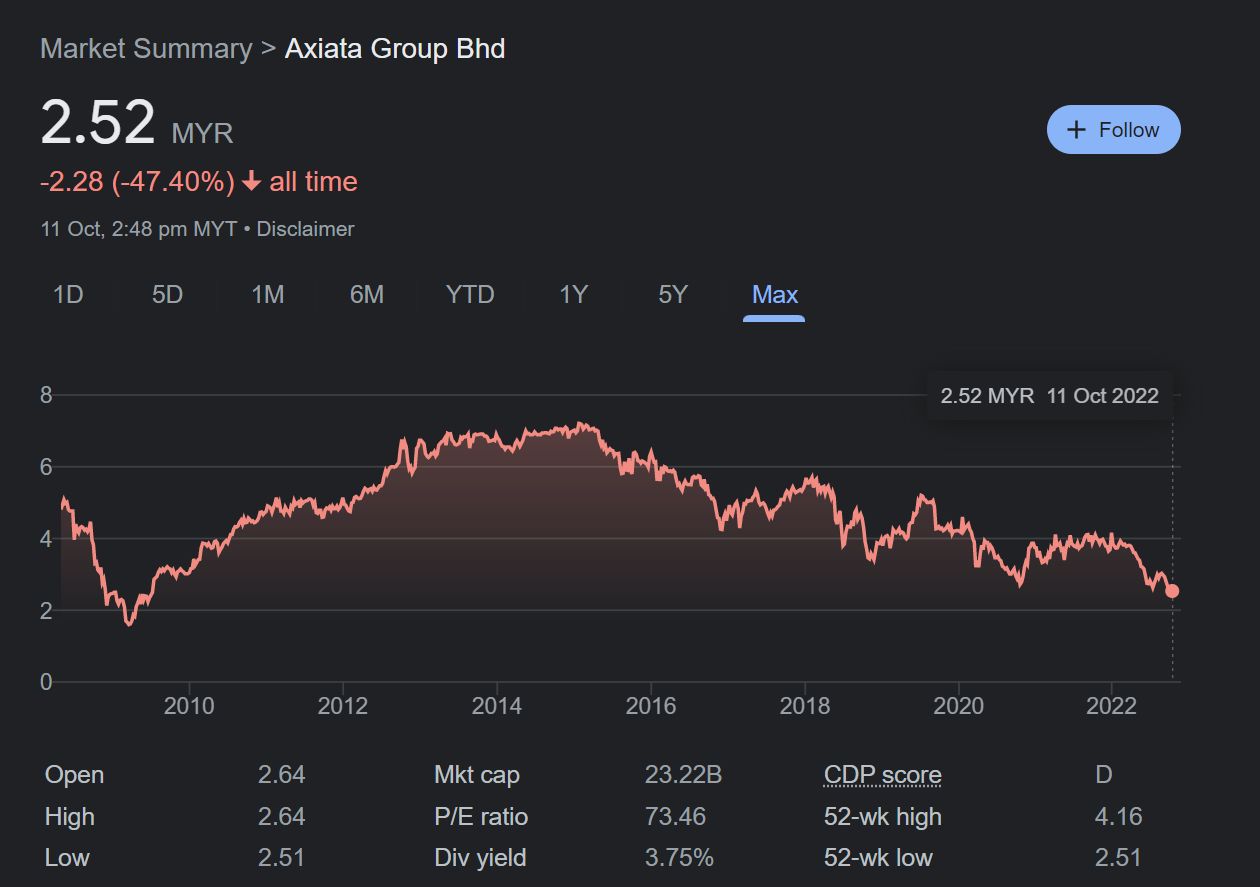This image displays a detailed market summary screen for the company "Exeata Group Bhd." The background is black, providing a stark contrast to the various text colors used. At the very top, the title "Market Summary" appears in gray, followed by a greater than symbol (">") and the company name "Exeata Group Bhd" in white.

The stock price is prominently displayed as "2.52 MYR," with a red downward indicator below it, showing a decrease of "-2.28" MYR (equivalent to -47.40%). This decline is illustrated with a downward-pointing arrow. To the right of this information, there is a blue "Follow" button for tracking the stock.

Beneath the stock price, the date and time are provided: "11th October, 2:48 PM MYT." A disclaimer follows this timestamp. The page also offers options to view the market summary over different time frames: 1 day, 5 days, 1 month, 6 months, year-to-date, 1 year, 5 years, and max.

A graph occupies the middle of the screen, visualizing the historical performance of the company's stock from 2010 to 2022. Below the graph, key metrics are listed:

- **Open:** 2.64 MYR
- **High:** 2.64 MYR
- **Low:** 2.51 MYR

To the right of these values, additional financial details are provided:

- **Market Cap:** 23.22 billion MYR
- **P/E Ratio:** 73.46
- **Div Yield:** 3.75%
- **CDP Score:** D
- **52-Week High:** 4.16 MYR
- **52-Week Low:** 2.51 MYR

These details collectively offer an in-depth overview of the financial standing and recent performance of Exeata Group Bhd.